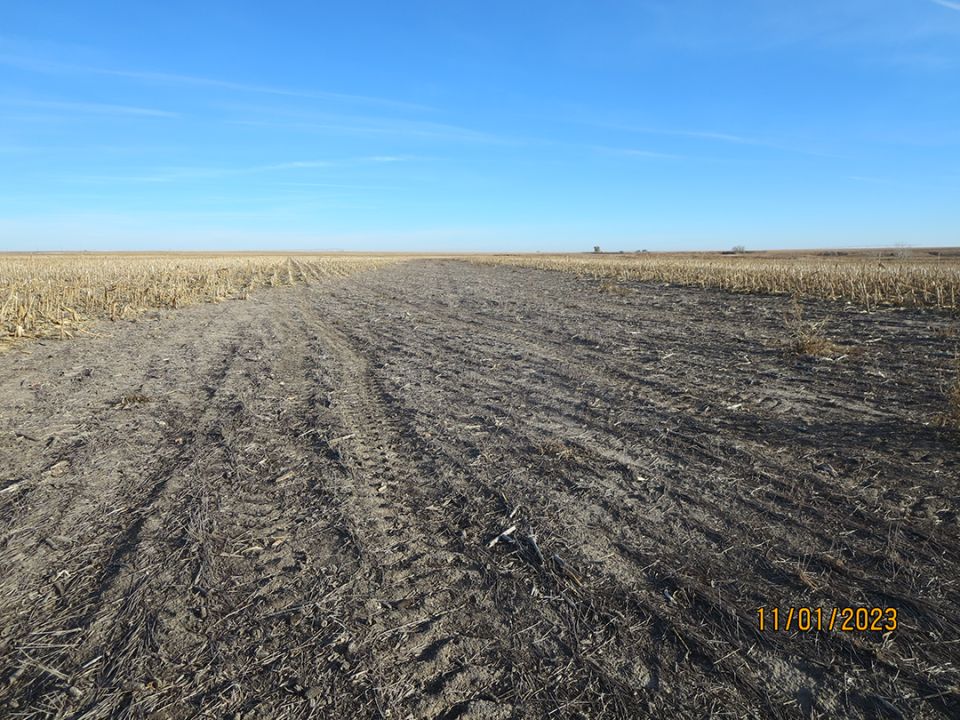This image depicts a vast, barren field under a bright blue sky, adorned with wispy streaks of clouds. The photo is timestamped with the date 11/01/2023 in orange letters in the lower right corner. The field stretches endlessly to the horizon, featuring predominantly dry, black dirt crisscrossed by numerous tire marks, suggesting that multiple vehicles have traversed the area. Off to the back left, there is a patch of yellowing, dry grass, and in the far distance, a tiny, barely discernible structure is visible. The overall appearance of the field is desolate, with a dry, almost matte texture and sparse, unhealthy-looking weeds scattered throughout.